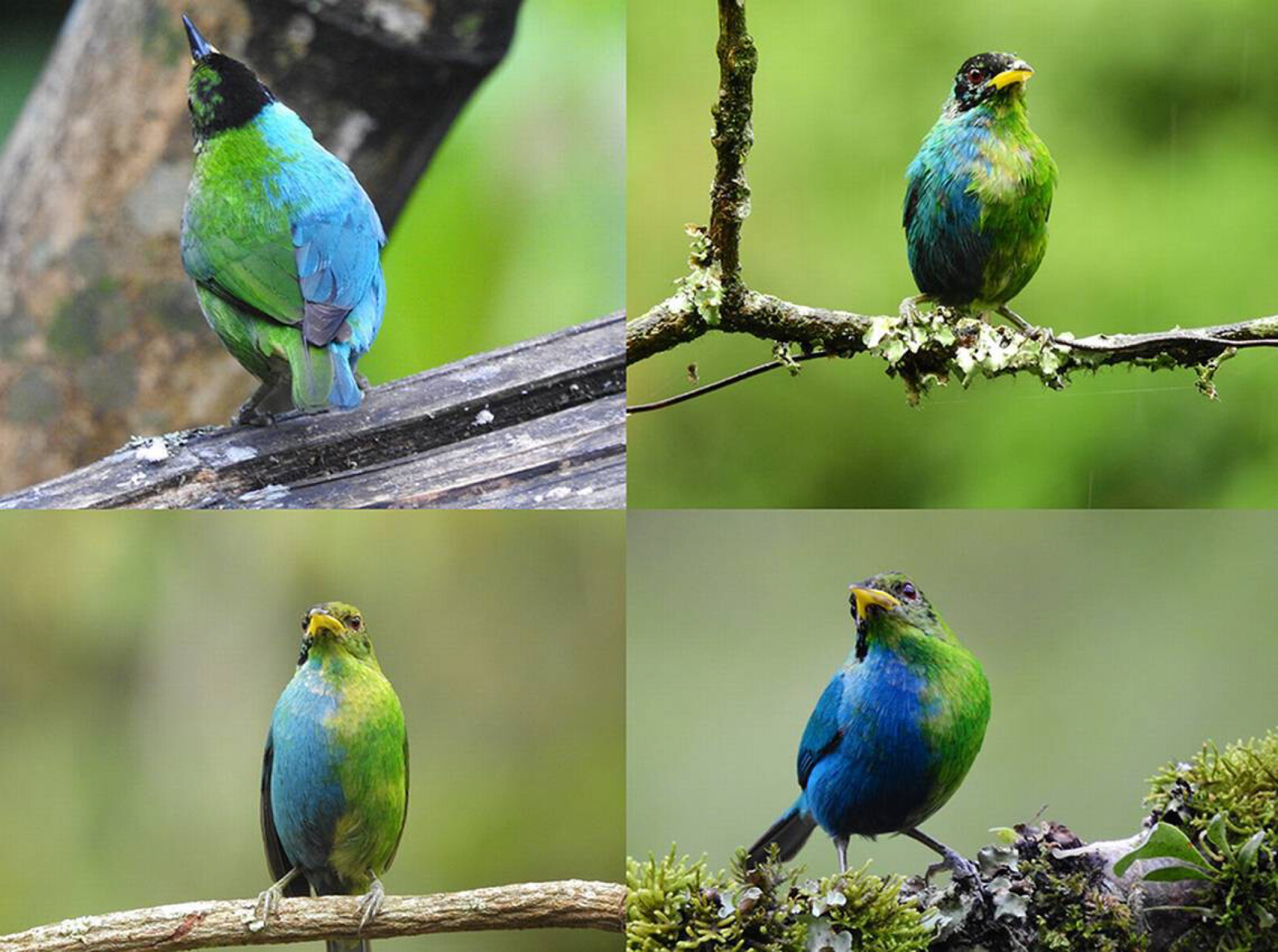The image is a collage featuring four photos of the same exotic bird, captured from different angles and perched on various branches. This eye-catching bird has a strikingly divided plumage, with the right side flaunting a deeper shade of blue, while the left side and back are a vibrant green. It also features a mix of blue and green tail feathers, a predominantly black head, and a distinctive yellow beak. 

In the first photo, located in the upper left panel, the bird is viewed from the back, sitting on a weathered wooden railing with a tree trunk in the background. The second photo, directly below, shows a frontal view of the bird on a different branch, emphasizing its unique coloration. The third panel, situated in the lower right, depicts a similar frontal angle but this time the bird appears to be holding a worm in its yellow beak, perched on a branch adorned with green sprouts. The final photo, in the upper right panel, also shows a frontal view of the bird, sitting on a moss-covered branch with a green backdrop, providing a slightly different perspective of its ruffled feathers. Each shot captures the bird's natural beauty and intricate feather patterns in a serene outdoor setting.